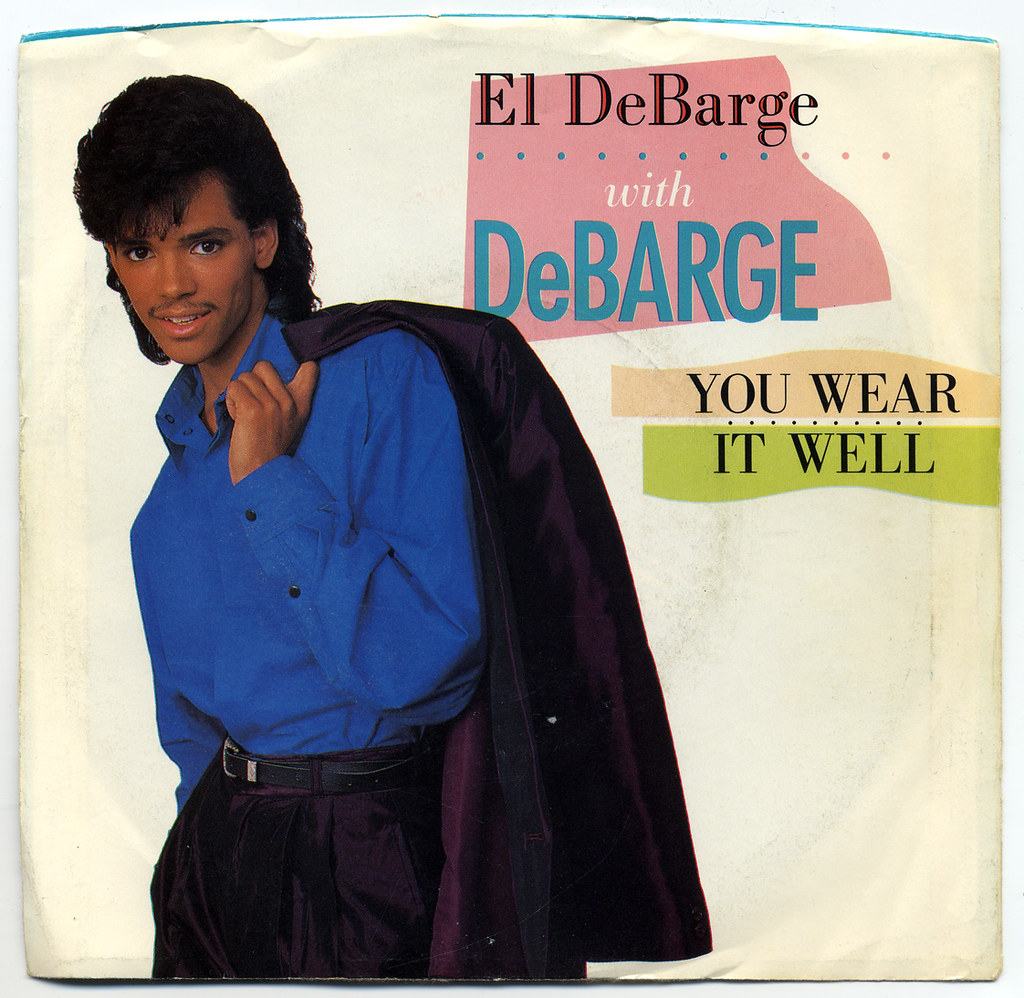The image is of a record cover featuring a young African-American gentleman posed against a cream-colored, slightly aged background. On the right side of the cover, the man, with medium-length shaggy black hair and brown eyes, gazes into the camera with a seductive smile. His ensemble includes a bright blue button-up shirt with black buttons unbuttoned at the top, tucked into black slacks or potentially purple trousers with a small black belt. Draped over his shoulder, held by his left arm, is a dark jacket with a purple lining, while his right arm hangs loosely at his side. Distinctive, colorful text to his right reads "El DeBarge with DeBarge" in a light pink square, followed by "You Wear It Well" displayed with parts in light brown, green, and teal hues, enhancing the vibrant aesthetic of the poster.